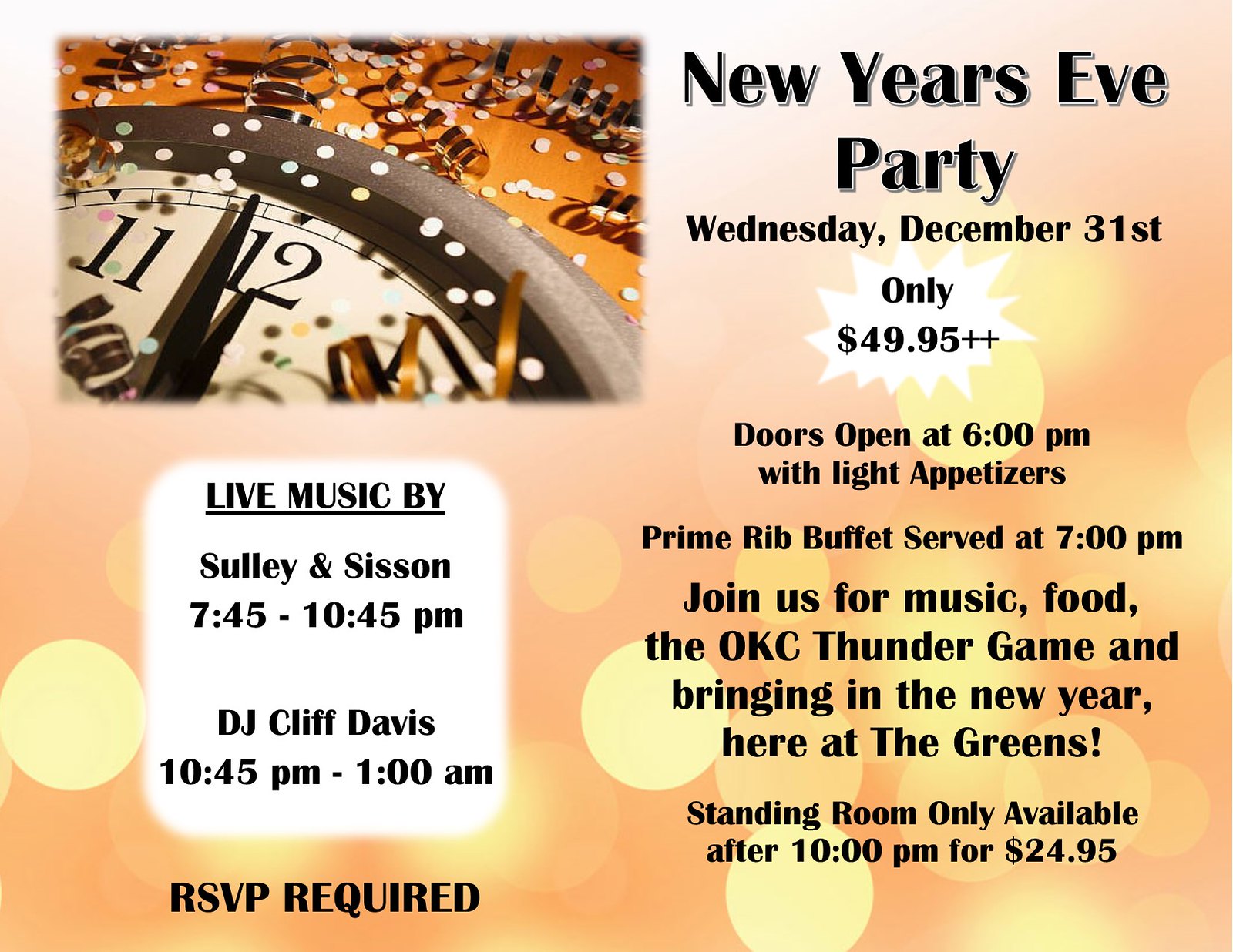The image is an advertisement for a New Year's Eve party, predominantly featuring orange, yellow, and white hues. On the top left, there is a partially visible clock moving towards 12, adorned with graffiti, streamers, and falling confetti, signaling the approaching New Year. The right side of the flyer prominently displays in bold, dark letters, "New Year's Eve Party, Wednesday, December 31st," with a ticket price of $49.95. Below this, it details the event schedule: doors open at 6 p.m. with light appetizers, followed by a prime rib buffet at 7 p.m. The event promises a night filled with music, food, the OKC Thunder Game, and festivities at the Greens. Standing room tickets are available for $24.95 after 10 p.m. A white box on the right lists the live music lineup featuring Sully and Sisson from 7:45 to 10:45 p.m., and DJ Cliff Davis from 10 p.m. to 1 a.m. At the bottom, it indicates that an RSVP is required to attend.